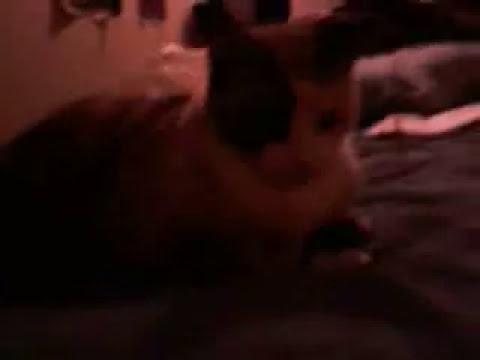This photograph captures a very blurry and underexposed image of a cat lying down, possibly on a blanket or a couch. Despite the poor lighting and shadowy composition, you can discern key features of the cat's appearance. The cat has a distinctive black patch over the right side of its face, extending to its ear, and a lighter patch on its left ear. Its fur transitions to a lighter color on the rest of its face and chest. The body of the cat seems to have varied color patterns, mostly dark with some lighter patches, particularly under its chin and underbelly. The background is also quite murky, but you can make out a light-colored wall with some pictures or items hanging on it, giving a hint of the setting. The bottom fourth of the image is almost entirely black due to lack of exposure, adding to the overall blurriness and difficulty in distinguishing finer details.